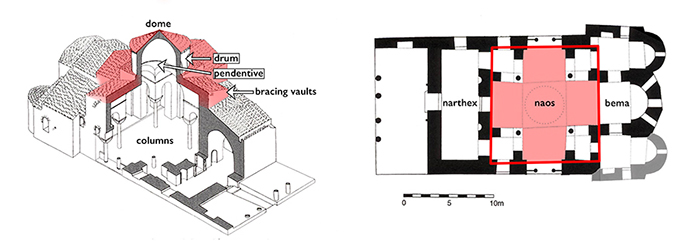This image features a detailed architectural diagram against a white background, showcasing two primary illustrations: a partial cutaway view of a house on the left and a floor plan on the right. The left side presents a 3-quarter view of the house, where a section has been cut away to expose both exterior and interior elements. Notable structural components are labeled, such as the dome at the top, the drum, and the pendentive (P-E-N-D-E-N-T-I-V-E) directed towards the middle of the house. Bracing vaults are also identified, with some highlighted in red, and central columns are distinctly marked in black. 

On the far right, the floor plan provides a top-down view of the house, illustrating the layout of rooms and structural features. It includes terms such as Northex, Naos (highlighted with a red square), and BEMA (B-E-M-A). A scale indicating 0 to 10 meters is positioned at the bottom for size reference. The correlation between the cutaway section and the floor plan is emphasized by the use of consistent red highlights, providing a clear visual connection between different perspectives of the house's architecture.